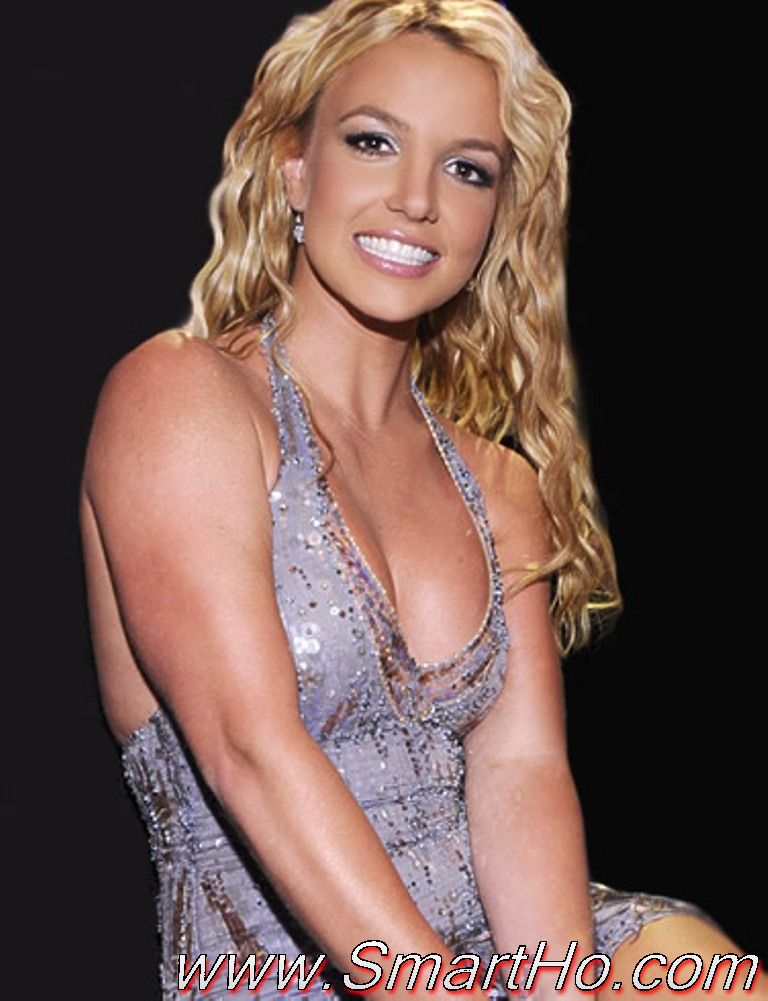The image features Britney Spears sitting down and facing the right, adorned in a stunning, low-cut, sleeveless, V-neck dress that sparkles with silver sequins and bedazzles. Her cleavage is prominently displayed. She is smiling broadly, showcasing her very white teeth, though her clenched jaw hints at a tense or forced expression. Her blonde, wavy hair cascades past her shoulders, nearly reaching her elbows. Britney's eye shadow is silver, her lips are painted a light pink, and she wears earrings that complement her glamorous appearance. Her toned legs are partially visible with the dress extending to her thigh, revealing above-the-knee coverage. The backdrop is entirely black, which contrasts sharply against the vibrant image of Britney and implies that she was cut out from a different background. At the bottom of the image, in white letters with a red shadow, the text reads "www.smarthoe.com."